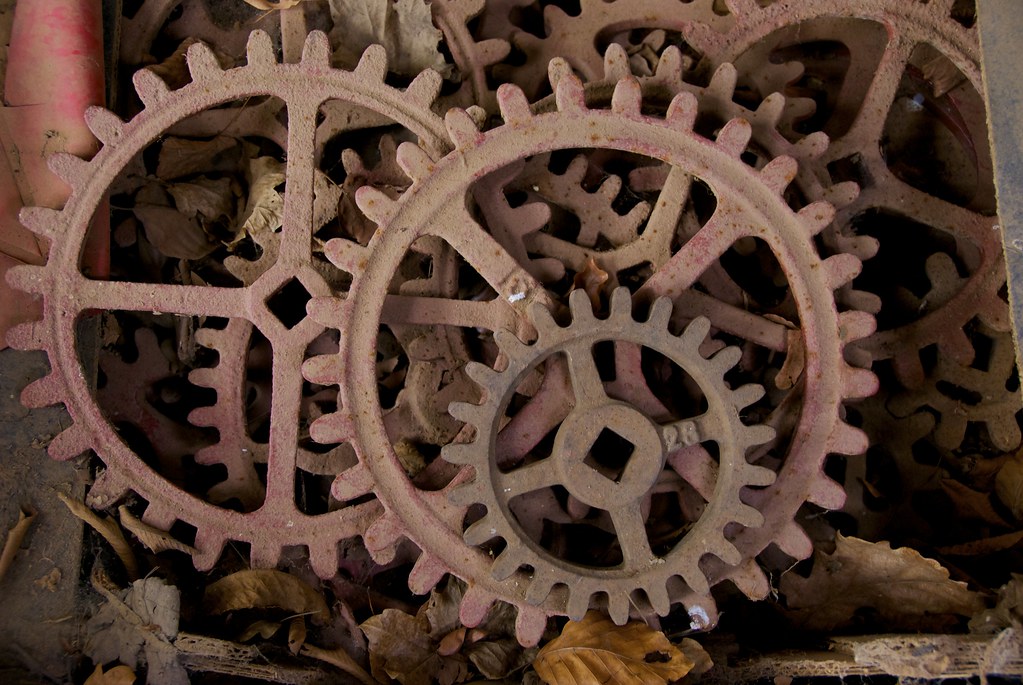The image captures an intricate assortment of gears arranged against an outdoor setting, scattered with leaves and rocks. In the foreground, two prominent gears with a distinctive pinkish-reddish hue draw immediate attention; these gears are large, with an abundance of teeth. The gear on the right bears the number "28" engraved on its side. Nestled between them, slightly below the pink-red gear to the right, lies a smaller grayish gear. Surrounding these principal gears are darker brown gears, creating a layered depth. To the top left of the image, a red object subtly adds to the industrial texture, while at the bottom of the frame, there is an orangish-copperish leaf and more leaves in the darker bottom right. Despite their intricate assembly, the gears appear unused, each featuring teeth on the outside and dual crossbars converging at the center, hinting at potential mechanical integration. The natural light illuminates the scene, enhancing the clarity and color of the image.